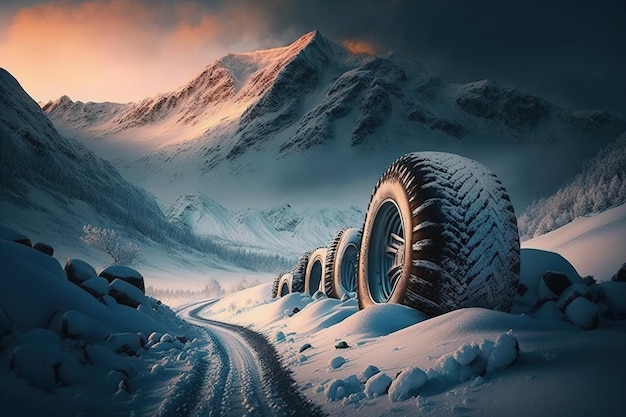This intricate painting depicts a winter scene with a long, snow-covered road leading into a mountainous landscape. In the distant background, a majestic, snow-capped mountain is illuminated with an orange haze, likely indicating a sunset, adding an amber glow to the tips of clouds in a dark grey, cloudy sky. In the foreground, the road is bordered by snow-covered terrain and dotted with small rocks. Prominently, four enormous, aggressive snow tires, each appearing to be about 20 feet high, are lined up along the side of the road. The tires are partially covered in snow, with snow accumulated on their treads and rims, suggesting recent use. Some trees are sparsely visible poking out from behind the tires. The painting effectively captures the serene yet somewhat surreal essence of a desolate, snow-filled valley transitioning towards a distant, luminescent mountain.